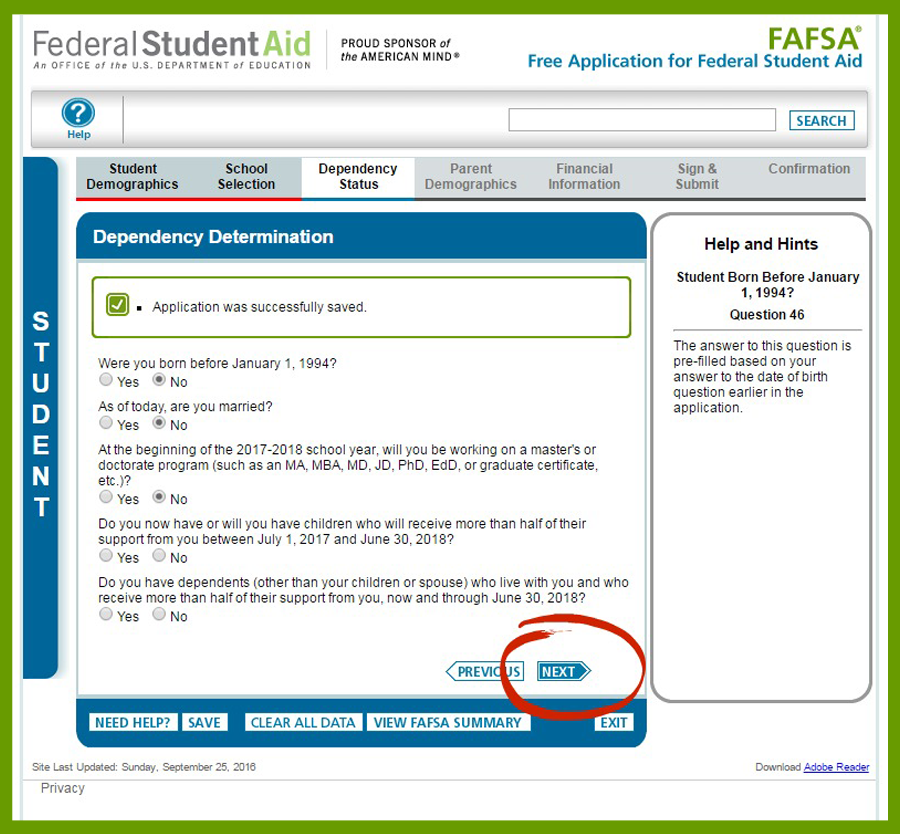The image features a white background framed by a dark green border. In the top left corner, there is text that reads "Federal Student Aid, an office of the U.S. Department of Education, proud sponsor of the American Mind." The main header says "FAFSA: Free Application for Federal Student Aid." Below the header is a gray box containing a blue circle with a question mark in the center, labeled "Help." To the right of this box, there is a search bar. 

Underneath, a series of clickable sections labeled "Student Demographics," "School Selection," "Dependency Status," "Parent Demographics," "Financial Information," "Sign and Submit," and "Confirmation" are listed. On the left side, a vertical blue box labeled "Student" runs up and down, while a horizontal blue box labeled "Dependency Determination" runs left to right, containing a series of questions. 

At the bottom of the image, there are navigation buttons – a "Previous" button on the left and a "Next" button on the right. The "Next" button has been circled conspicuously in red, indicating that it has been edited to draw attention.